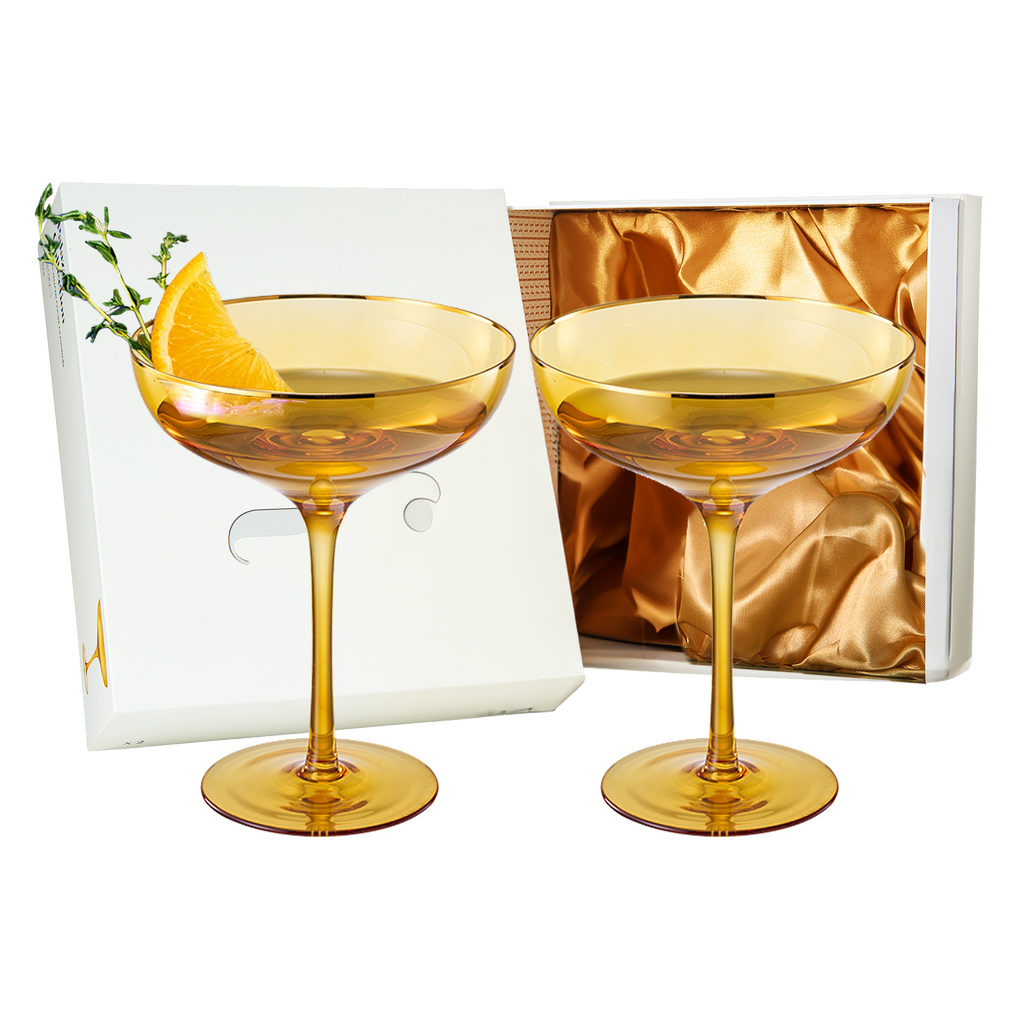The image features two amber-colored champagne coupe glasses, each containing a small amount of liquid, likely a cocktail. The glass on the left is adorned with a sprig of rosemary and an orange wedge, while the glass on the right is left without any garnish. Both glasses are side by side against a backdrop that includes an open white box with a gold silk-like interior, suggesting the glasses might have originally been packaged inside it. The lid of the box is off to the side, and the glass with the orange garnish stands in front of the white box with its luxurious gold lining. This setup, paired with the champagne coupes and their upscale presentation, gives the impression the image may be part of an advertisement or promotional material for these elegant drinking glasses.